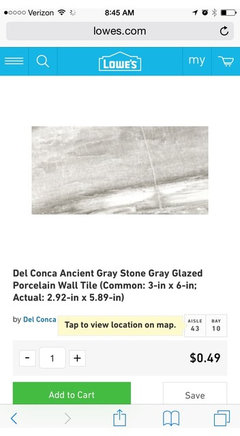A detailed view of a smartphone screenshot displaying various interface elements and information. 

At the top of the screen, the status bar has a white background. It features five circular indicators, where four are white with black outlines and one is solid black. The carrier name, "Verizon," is displayed next to "Verizon Wireless," followed by Wi-Fi signal bars indicating a strong connection.

In the center of the status bar, the time "8:45 a.m." is prominently shown in black text, labeled as "NASA time." Adjacent to the time is a black alarm clock icon with an arrow pointing diagonally to the right side. The battery icon shows less than 50% remaining, with the filled portion in black.

Below the status bar, the screen is divided into sections. The top part features a web browser interface with a gray and black theme. The URL bar displays "Lowes.com" along with a black refresh button shaped like a nearly complete circle. Adjacent to it is a light blue rectangle with a white magnifying glass icon, indicating a search function, and three horizontal white lines symbolizing a menu. The text "Lowe's" appears in white next to a house icon, followed by "Mine" and a shopping cart icon, both in white.

Beneath this, the product details are visible on a white background. A grayish-white stone texture serves as the backdrop for the text. In black text, the product is described as "Del Connor Asian Graystone Gray Glaze Porcelain Wall Tile." Further details include "Proceed common... 3-inch by 6-inch... actual... 2.92-in by 5.89-in" by Del Connor. A prompt to "tab to view location on map" follows. The price is listed as "$0.496" per tile.